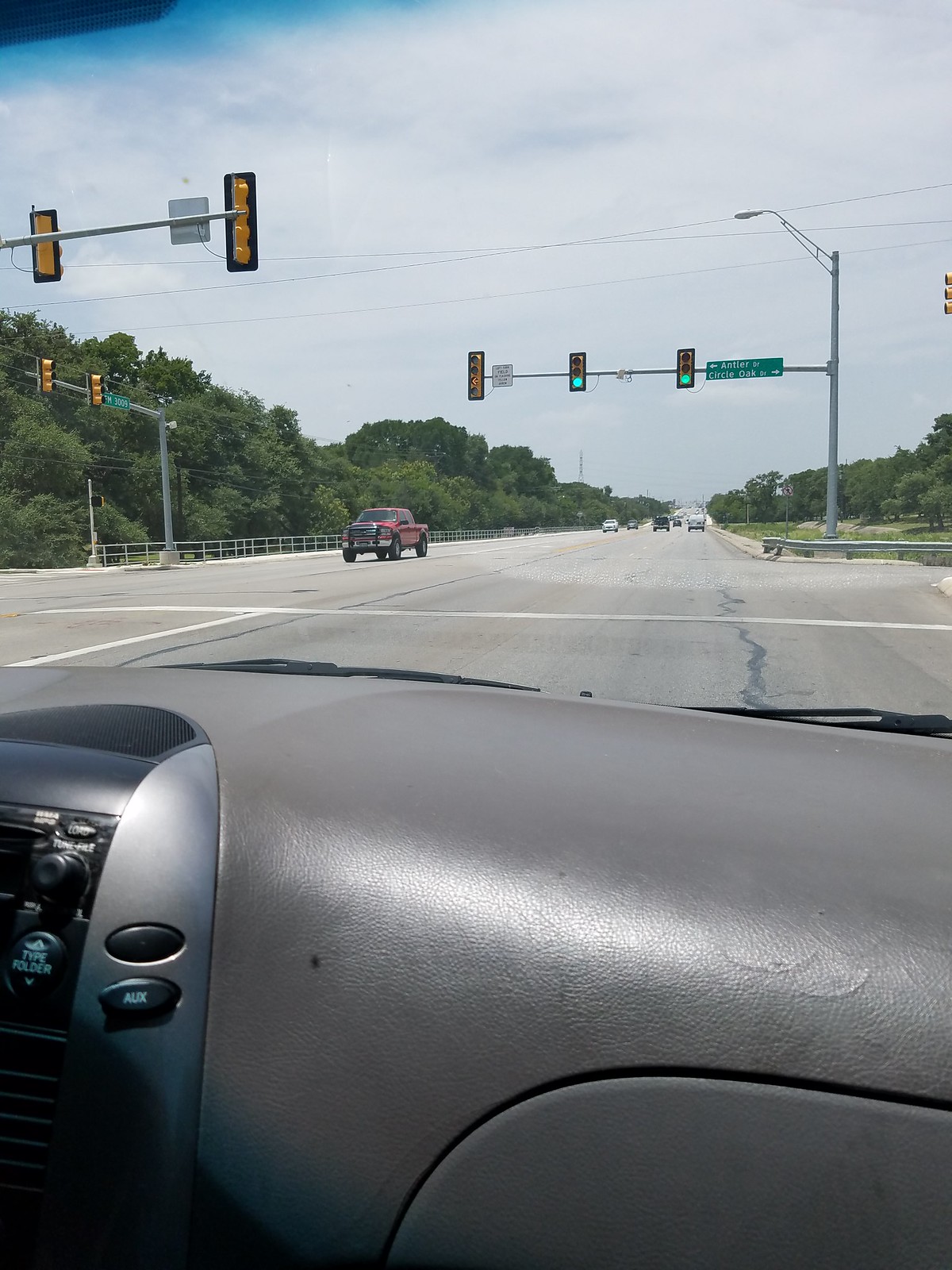This point-of-view photograph, likely taken from the passenger side of a vehicle, provides a vivid scene viewed through the windshield. The foreground features a grayish plastic dashboard reflecting some light, with visible knobs on the center console, one labeled "AUX" for auxiliary input. Beyond the dashboard, a road stretches into the horizon at a T-shaped intersection, flanked by trees on both sides—denser on the left and sparser on the right. The traffic light ahead shows green, and a red pickup truck approaches from the opposite side. Accompanying the green lights are two additional green signals, and a horizontal green road sign is affixed to a tall aluminum light pole meant for illuminating the road. In the distance, more vehicles head toward the horizon, adding depth to the scene.